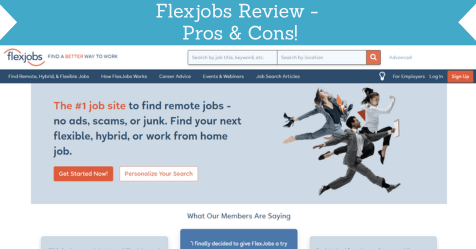The image features a prominently placed blue banner at the top with bold white text stating, "FlexJobs Review - Pros and Cons." Below this banner, two open fields are displayed side by side. On the right field, there's an orange button with a white magnifying glass icon. The left field showcases the FlexJobs logo in blue, accompanied by an orange line curling around it, with the slogan "Find a Better Way to Work," where the word "Better" is highlighted in orange.

A blue navigation strip runs below these fields, containing various sections related to job searches and career resources. Despite the low resolution making the text somewhat difficult to read, the sections appear to include "Find Remote, Hybrid, and Flexible Jobs," "Flexible Job Works," "Career Advice," "Events and Webinars," and "Job Search Articles." On the right side of the navigation strip, there are links for "For Employers," "Login," and an orange "Sign Up" button.

Following the navigation strip, there's an image depicting three people—two women and a man—jumping in the air while dressed in business attire. This image is accompanied by the text, "The #1 Job Site to Find Remote Jobs - No Ads, Scams, or Junk. Find Your Next Flexible, Hybrid, or Work from Home Job." Below this, two buttons are visible: an orange "Get Started" button and a white "Personalize Your Search" button. At the very bottom of the image, there's text reading, "What Our Members Are Saying."